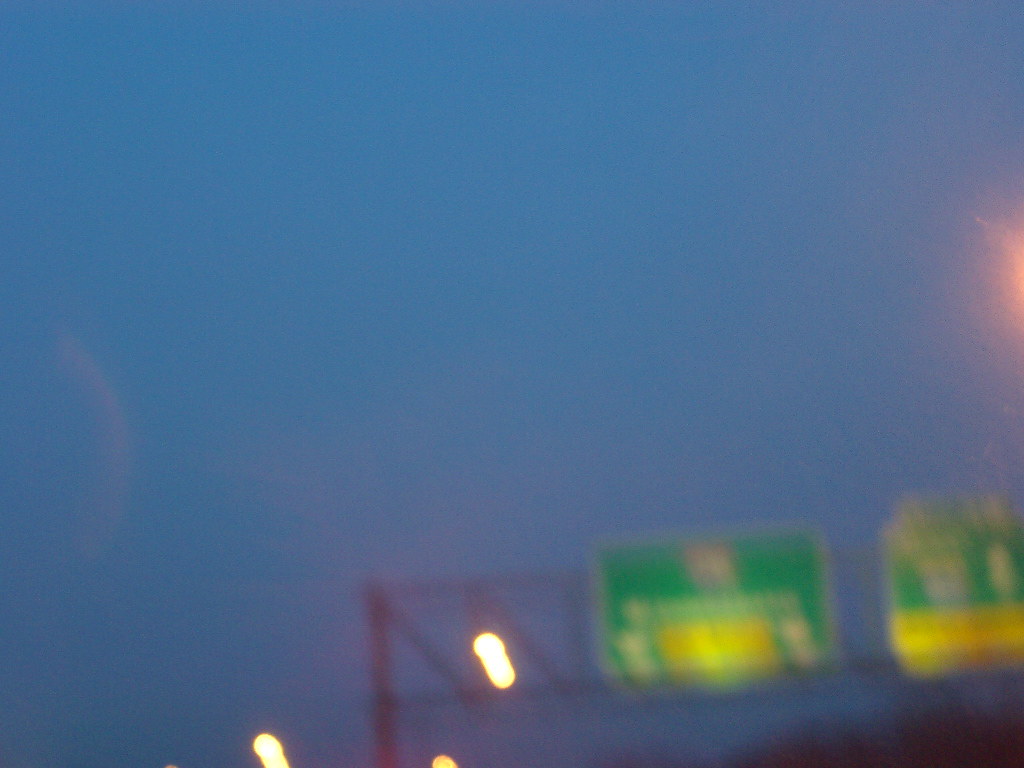This image captures a scene likely taken during either early morning or early evening, as suggested by the dim natural light. The sky exhibits a clear blue hue with no clouds, enhancing the serene yet somewhat mysterious atmosphere. Dominating the frame are large interstate signs suspended by a broad metal bar. Among these signs, the distinctive red, white, and blue interstate shield can be identified, framed by yellow tips which indicate 'Exit Only' lanes. The signs are flanked by several blurred light fixtures, possibly three or four, their details obscured due to motion or a slight camera shake. On the right side of the image, about two-thirds up, a soft glow hints at the presence of a street light. The overall composition leaves the exact location ambiguous, as the viewer's perspective is focused upwards, providing an isolated view of the signs against the tranquil sky.